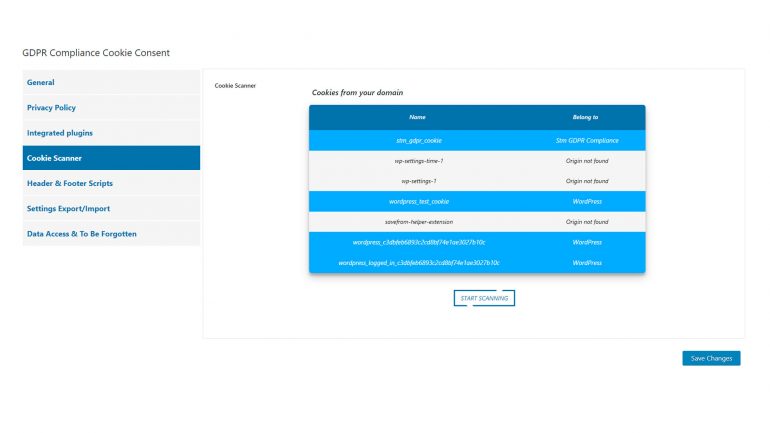The image is a screenshot featuring a toolkit for GDPR compliance with a white background. The main interface highlights various functionalities such as cookie consent, general privacy policy, integrated plug-ins, and a cookie scanner. The interface is neatly organized with several sections, each delineated by headers and footers in dark blue rectangles. 

Key elements include:

1. GDPR Compliance and Cookie Consent: A dedicated section likely providing tools and settings for managing user consents in accordance with GDPR regulations.
2. General Privacy Policy: A segment probably aimed at offering templates or guidelines for creating privacy policies.
3. Integrated Plug-ins: This section suggests the availability of plug-ins to seamlessly integrate with existing systems.
4. Cookie Scanner: Twice mentioned, this scanner presumably identifies and categorizes cookies present on the user's domain.

A special feature of the screenshot is an ordered list with alternating blue and white backgrounds for each item:
1. The first item is highlighted in a blue rectangle.
2. The second and third items are in white rectangles.
3. The fourth item again is in a blue rectangle.
4. The fifth item reverts to a white rectangle.
5. The sixth and seventh items are back in blue rectangles.

At the bottom of the interface, a large blue rectangle contains the text "Start Scanning," inviting the user to initiate the cookie scanning process.

One item in the list is partially obscured, possibly containing a word starting with 'A'. The structured layout and organized sections of the interface enhance user navigation and comprehension of the provided tools for GDPR compliance and cookie management.